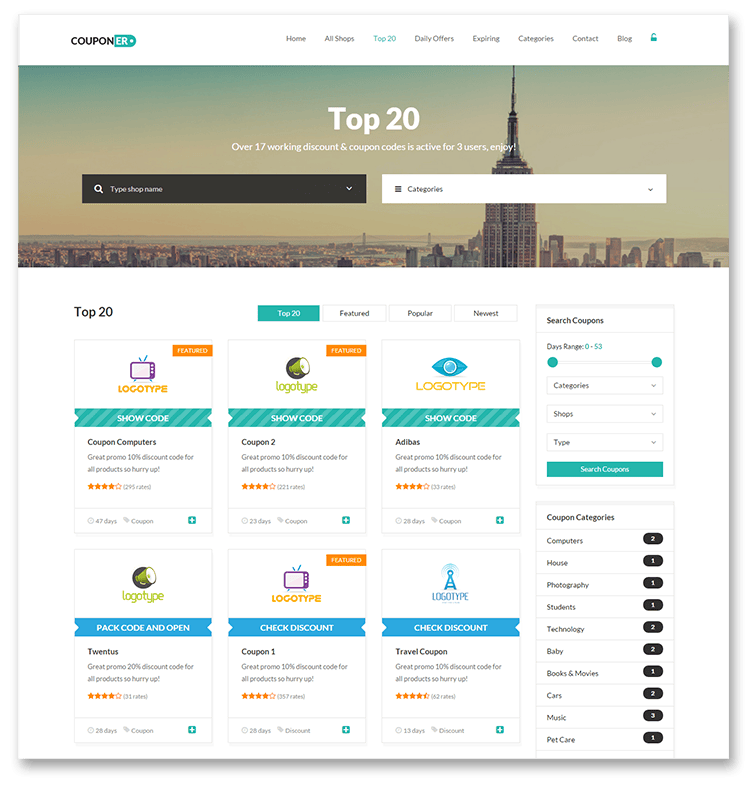The website screenshot features a clean and structured layout with a prominent white banner at the top. The banner includes navigation options on the far left: "Coupon ER," "Home," "All Shops," and "Top 20," outlined for emphasis. Adjacent to these options are additional links: "Daily Offers," "Expiring," "Categories," "Contact," and "Blog."

Below the banner, the background showcases a city skyline with a very tall skyscraper set against a bluish-gray sky. The text "Top 20" is prominently displayed, indicating the section being viewed. Accompanying this, it notes, "Over 17 working discount and coupon codes are active for 3 users. Enjoy."

The center of the page features two search bars; the left one is black with the placeholder text "Type Shop Name," while the right one is white with "Categories" as the placeholder. Navigation tabs below these search bars include "Top 20," "Featured," "Popular," and "Newest," with "Top 20" currently selected.

Beneath this, highlighted deals are presented with distinctive blue logotype icons and "Show Code" buttons. Each listing includes a promotion description: "Great Promo, 10% Discount Code for all products," a sense of urgency with "Hurry Up," and an average rating of 4 out of 5 stars. Brands like "Coupon Computers," "Coupon 2," "Adibus," and various other promotional codes follow this format consistently.

To the right, a vertical menu offers additional navigation, including "Search Coupons," a days range slider from 0 to 53, categories, and shops filters. Listed coupon categories encompass a wide array of interests, such as "Computers," "House," "Photography," "Students," "Technology," "Baby," "Books and Movies," "Cars," "Music," and "Pet Care."

By providing clear organization and multiple filters, this website aids users efficiently in finding the best coupon deals across various categories.